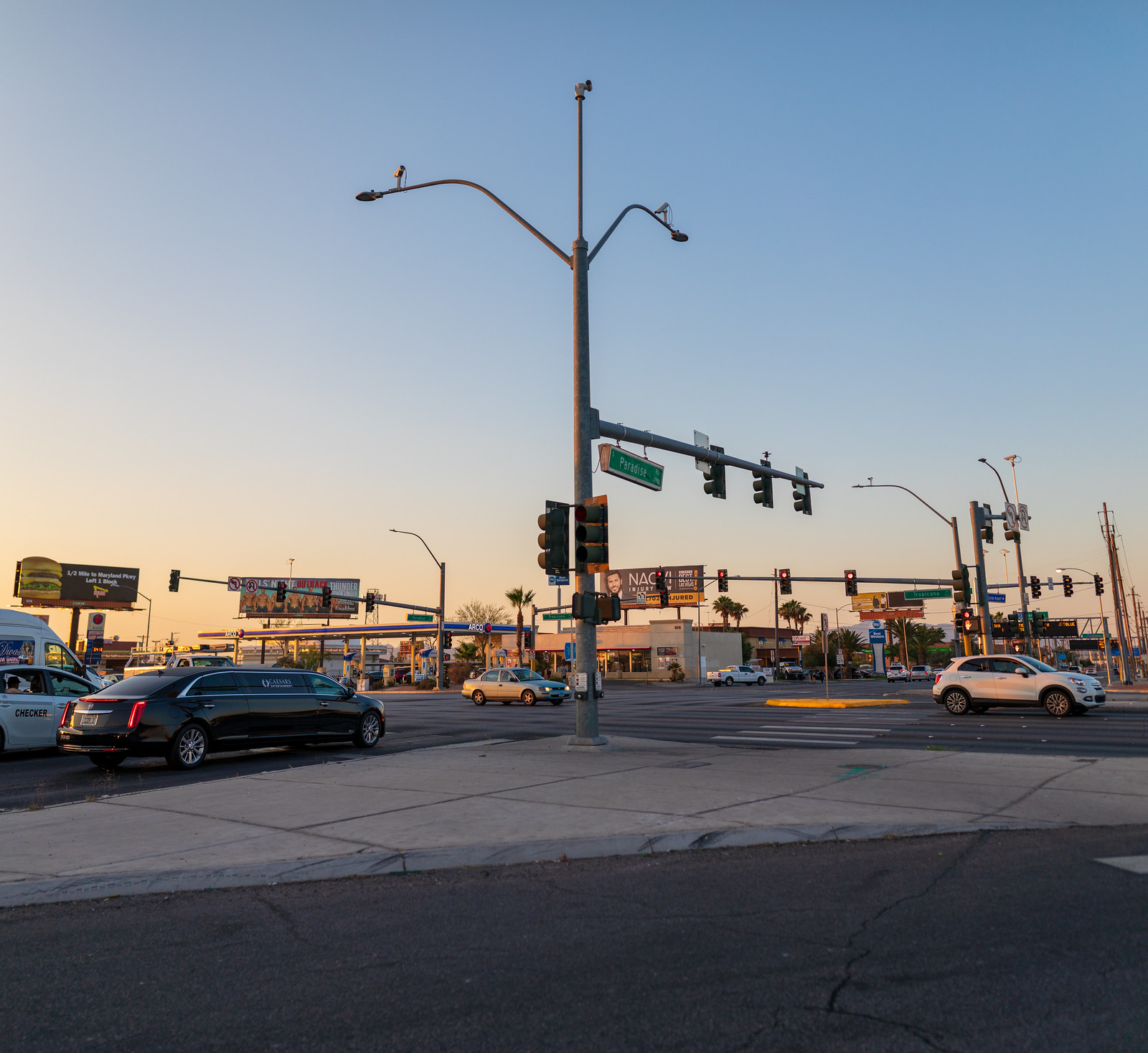A bustling intersection of two major roads captured from the perspective of a vehicle paused at a designated right-turn ramp. The expansive intersection features multiple lanes in both directions. Each corner is equipped with poles supporting street lights and what appear to be traffic cameras, along with traffic signals regulating the flow of vehicles. Diagonally across the intersection, an established gas station with an associated mini-mart is clearly visible.

To the right, a sleek black Cadillac stretch limousine stands out amongst the traffic, accompanied by a white car marked with "Checker" on its passenger door, likely signifying a checkered cab, and a white panel truck. Overhead, a collection of at least four elevated billboards dominates the scene from the distance. The leftmost billboard showcases a tantalizing image of a tall hamburger with a meat patty, cheese, and lettuce. The adjacent billboard appears to feature a series of images of a woman in a black dress. Another billboard carries an image of a person along with partially obscured text that reads "NAC." The other billboards and possible dealerships in the vicinity remain indistinct due to their distance and the angle of view.

The imagery depicted in the billboards and the varied vehicles contribute to the dynamic and busy atmosphere of this urban intersection.